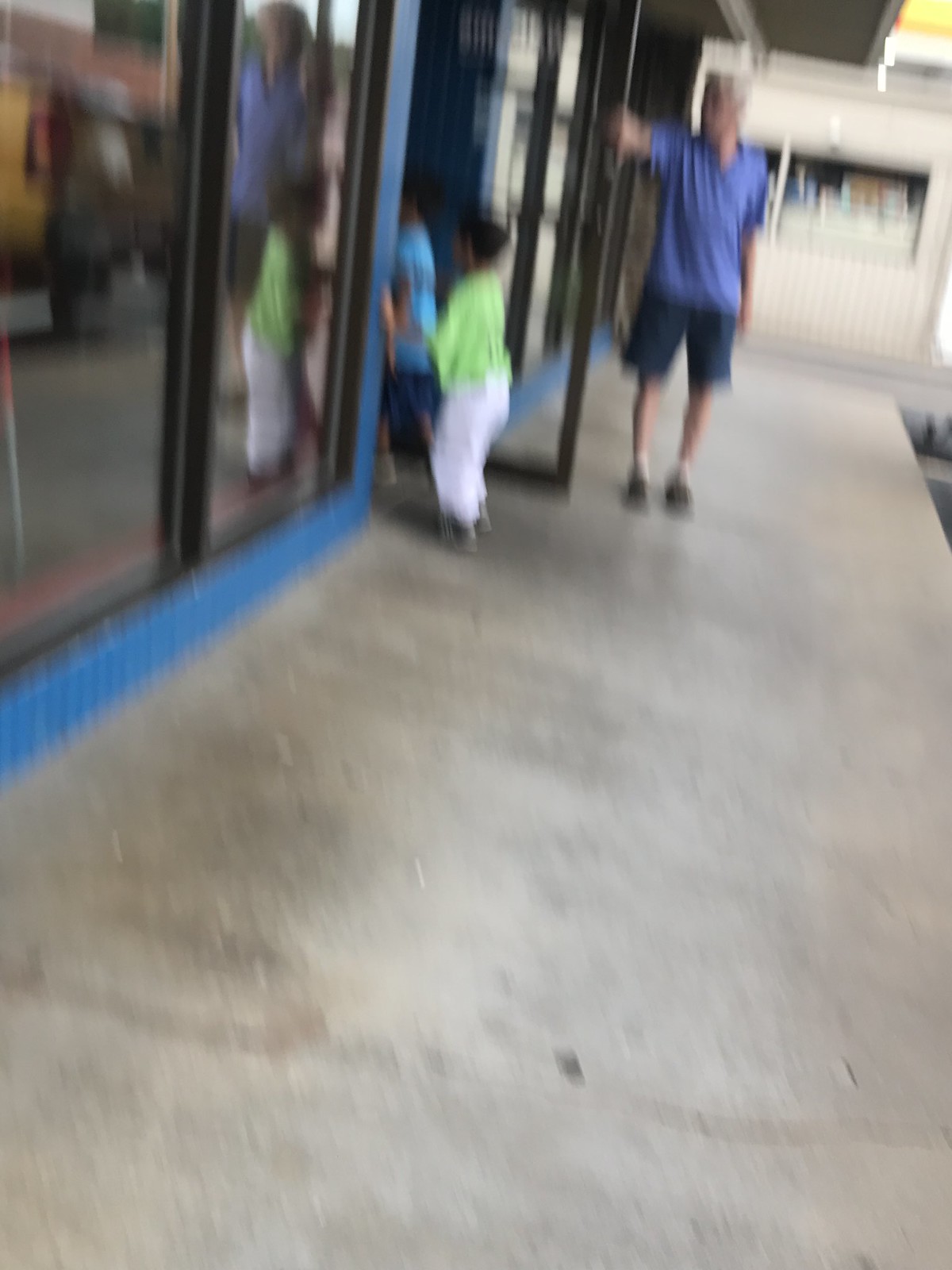In this blurry, out-of-focus image, a man with gray hair is seen holding a door open for two young children. The man, dressed in blue shorts and a matching blue shirt, stands on a cement walkway facing the camera. One child, wearing white pants and a green shirt, and with brown hair, is almost fully inside the building. The other child, also with brown hair, is dressed in blue shorts and a blue shirt, and is about to step through the doorway. The details of their faces and clothing are indistinct due to the blurriness of the photo. The setting appears to be the entrance to an unspecified building, and one of the reflective windows faintly captures the surrounding scene.